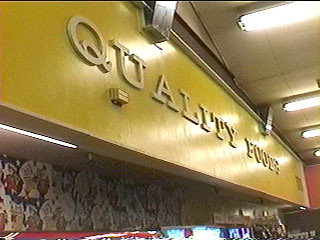The image is a square, somewhat aged photograph showcasing the interior of a store with a prominent sign. The sign, set against a bright yellow-gold, mustard-colored rectangular banner, features large, uppercase white letters that read "QUALITY FOODS," with notably wide spacing between each letter. This sign is affixed to the ceiling with metallic clips, beneath heavy-duty fluorescent lights embedded in a large tiled ceiling. 

To the right of the banner, there is a red header that likely indicates another section of the store, though the details are indistinct. Below the banner, the image captures a glimpse of blotchy wallpaper with white symbols on a black background and sections of a rusty orange wall. At the bottom, there's a vague outline of various hanging items, perhaps indicating additional food sections, but the specifics are unclear. The image aims upwards, making it challenging to discern the exact contents or layout of the lower shelves and counters.